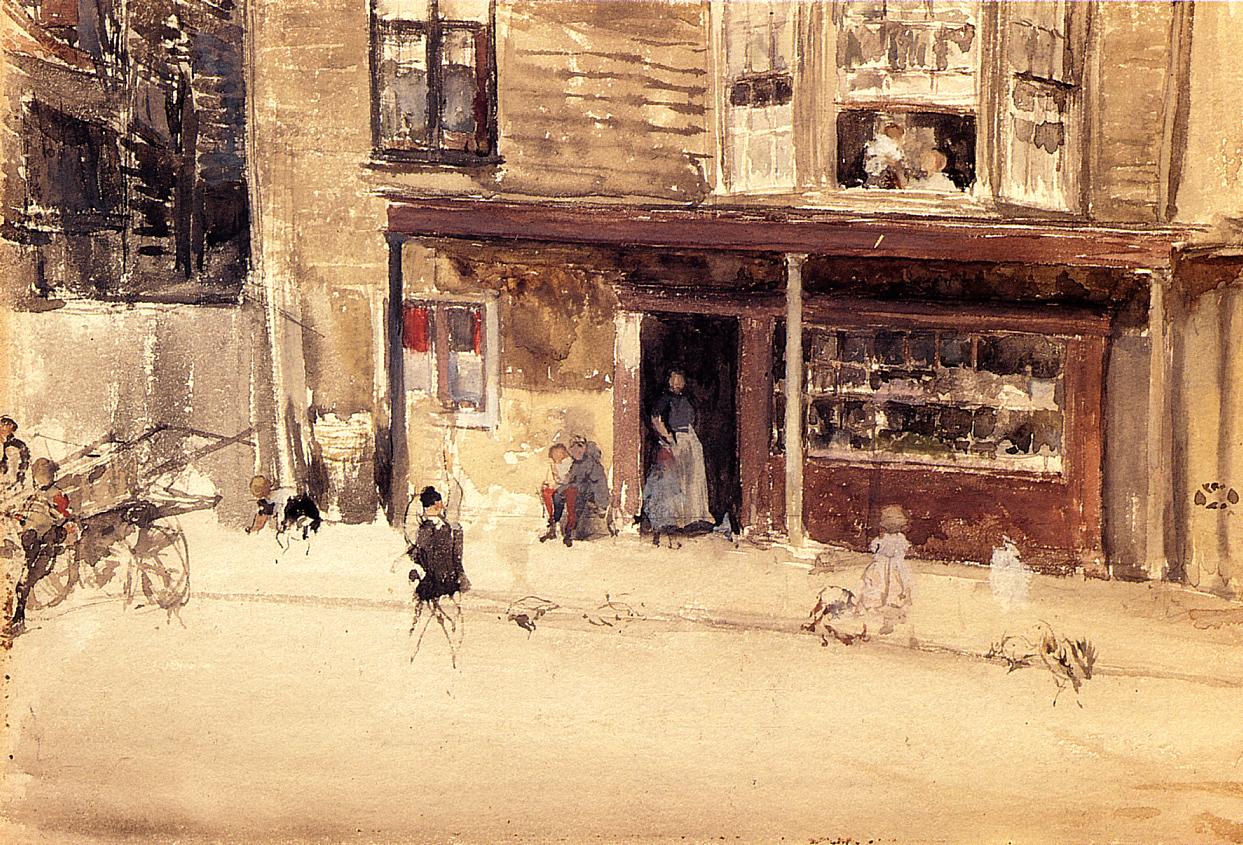This painting captures a bustling storefront scene with an impressionistic touch, characterized by earthy tones like beige, brown, and rusty hues. The structure, which has a distinctly Western American feel, features two stories. The upper floor has two windows – one open, revealing children playing inside, and a bay window where someone, possibly holding a child, is seated. The first floor, detailed with wood support beams and an overhang, contains a doorway where a woman in a white skirt and black jacket or apron stands blurred in silhouette. Nearby, a man sits on a bench with a child in his arms, possibly engaging in conversation with her. The scene extends to the foreground where people, including children, are either walking along the sidewalk or playing in the street. Additional activity is depicted with a wagon placed in front of the store, suggesting an ongoing unloading process. The painting, done in watercolor, combines loose brushstrokes that dissolve up close but coalesce into a detailed depiction when viewed from a distance.